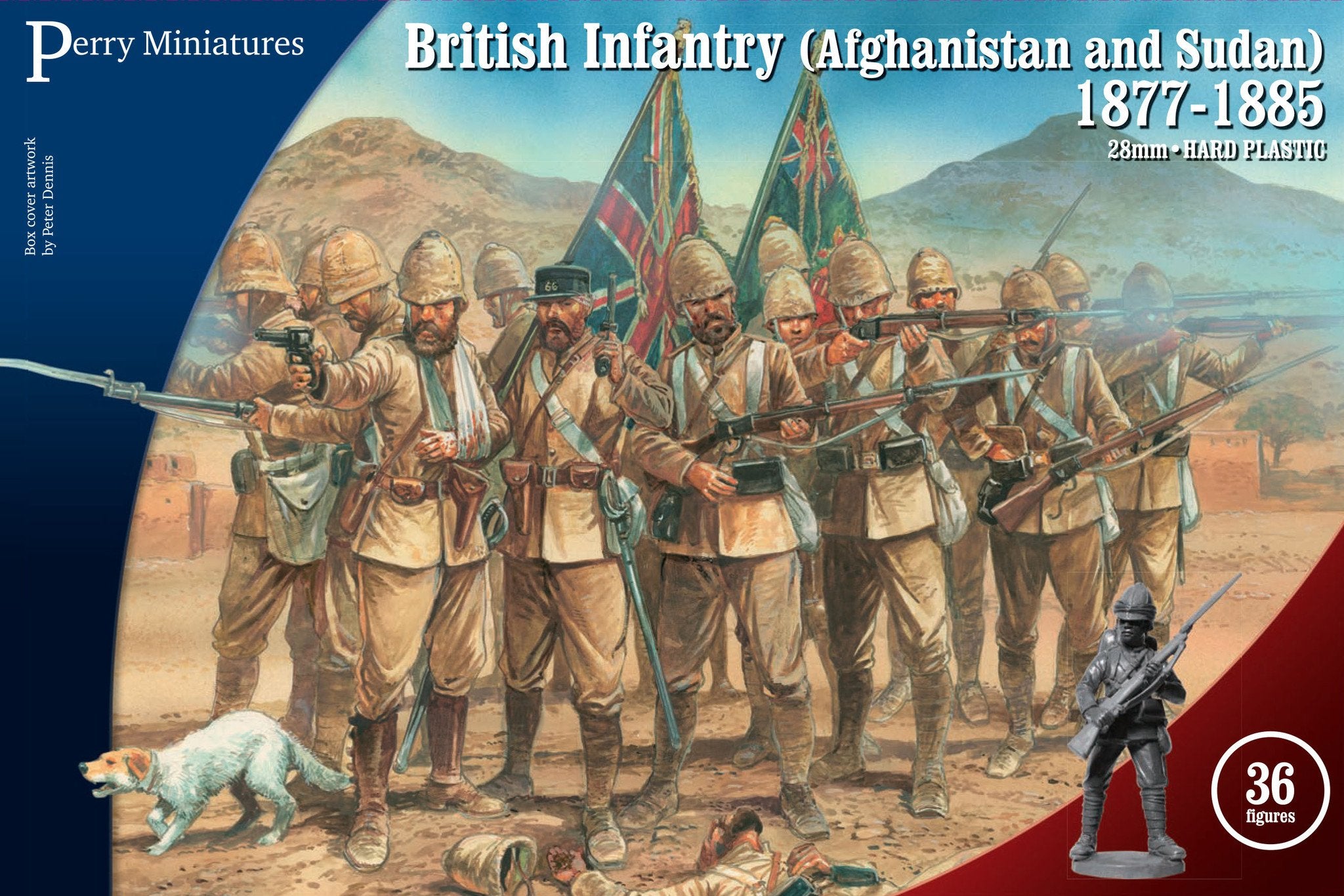The image is a detailed package cover for Perry Miniatures. It prominently features "British Infantry in Afghanistan and Sudan, 1877 to 1885" written in white in the upper right corner against a blue sky backdrop, along with "28mm Hard Plastic" indicating the figure size. The box's artwork is created by Peter Dennis and features brown-uniformed soldiers with helmets and boots, some holding rifles with straps and muskets. The upper left shows the Perry Miniatures logo in white on a dark blue half-circle. The bottom right includes a red section with the text "36 figures" in a white circle. The background displays mountains and a clear blue sky, with both British and Australian flags visible, adding to the historical context. A gray military figurine is showcased in the bottom right corner, emphasizing the intricate details of the figures included in the set.